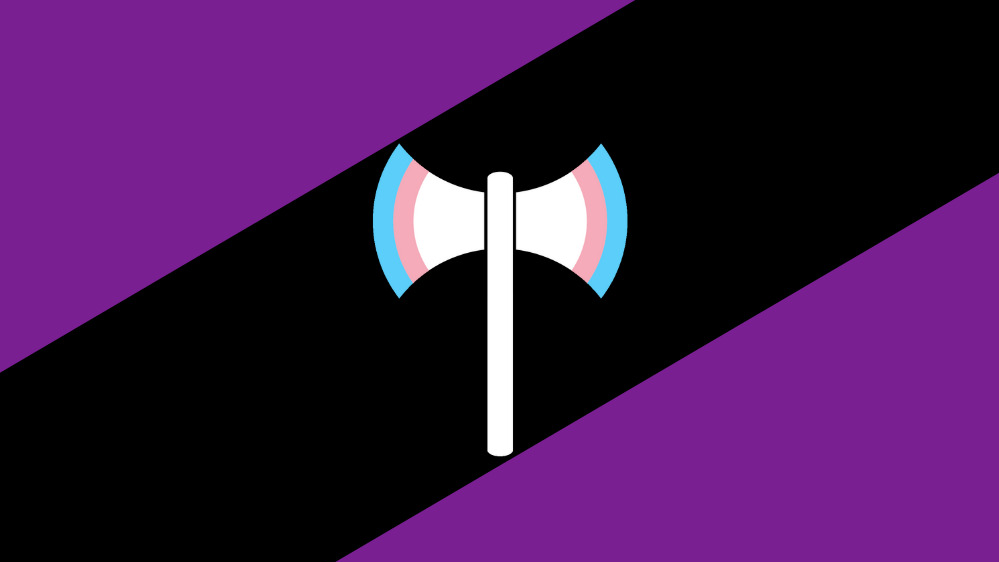The image is a simple, computer-rendered graphic featuring a white, double-headed axe centrally positioned. The axe blades are detailed with light blue and light pink stripes along their edges, reminiscent of pride flags associated with minor attracted persons. The axe is superimposed over a diagonal black stripe that cuts through the center of a rectangular background. The upper left and lower right corners of the rectangle are purple, forming triangular sections at either end of the black stripe. The image is a 2D design with no three-dimensional features and includes no text, highlighting its minimalist style.